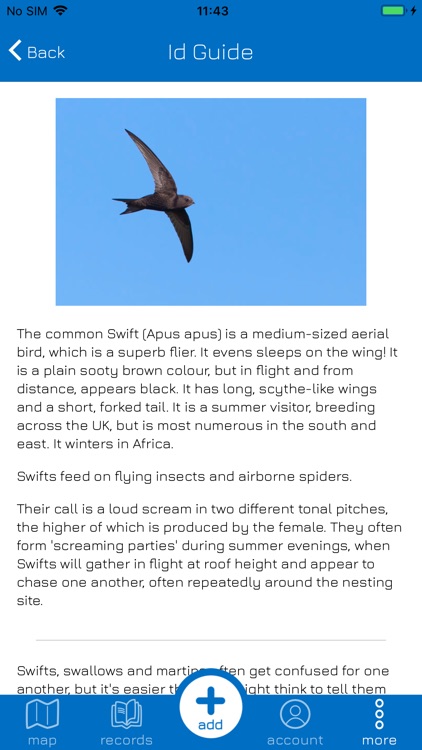A screenshot of a phone display is prominently shown. At the top of the screen, there is a dark blue border containing various icons: on the upper left, "No SIM" is indicated; the time "11:43" is displayed in the center; and a green battery icon is visible on the far right. Below this section, there is a back button on the bottom left, and centered text that reads "ID guide." 

The main content area features a white background divided by an image and text. The image, located at the top, captures a blue sky with a gray bird flying with its wings spread wide. This bird is identified as a Common Swift. 

The accompanying text provides detailed information about the Common Swift (Apis). It is described as a medium-sized aerial bird renowned for its flying prowess, even capable of sleeping while in flight. The bird is primarily a plain, sooty brown color but appears black when observed in flight from a distance. Its notable physical characteristics include long, scythe-like wings and a short forked tail. The Common Swift is a summer visitor to the UK, predominantly found in the south and east, and migrates to Africa for the winter. The bird's diet consists of flying insects and airborne spiders. 

Additionally, it is noted that the Swift's call is characterized by a loud scream in two tonal pitches, with the higher pitch being produced by the female. During summer evenings, these birds often engage in "screaming parties," where they gather in flight at roof height, chasing each other around their nesting sites.

At the bottom of the screen, there is another blue border featuring a circle in the center with a blue plus sign labeled "Add."